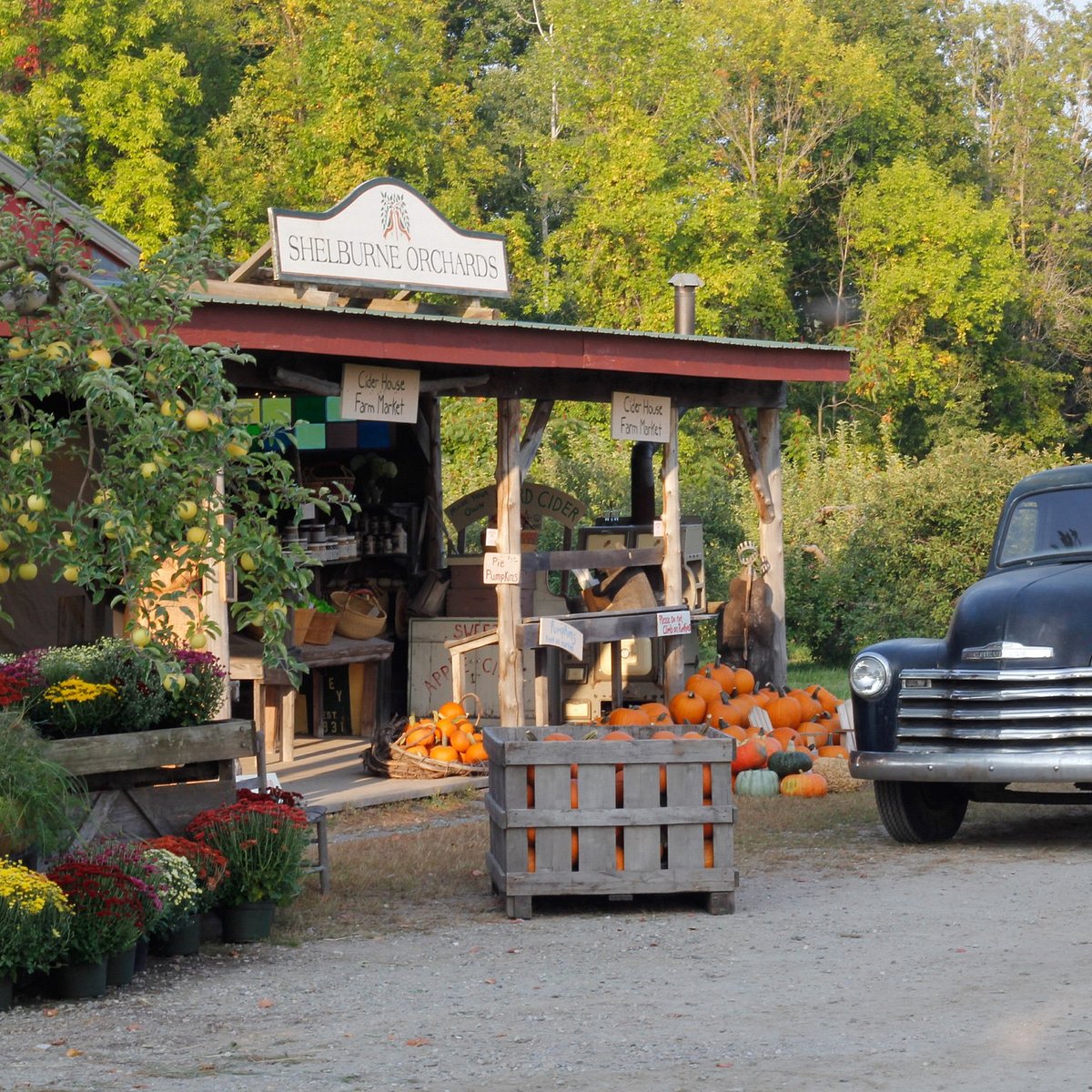The image depicts a quaint roadside market reminiscent of those found in rural Appalachia. Central to the scene is a charming, rustic stand with a red-trimmed tin roof and wooden pillars supporting an awning. The stand displays an assortment of pumpkins, both piled on the ground and neatly arranged in baskets and crates. Above the porch, a sign with a laurel logo reads "Shelburne Orchards," and another sign hanging from the awning announces "Cider House Farm Market." The surroundings are filled with vibrant flowering potted plants and additional produce, including what appears to be a pear tree laden with fruit. To the right of the market, a vintage black 1950s car with chrome grilles is parked, adding a nostalgic touch to the modern photograph. The scene is framed by a gravel driveway and lush trees, encapsulating the serene atmosphere of a disappearing American tradition.